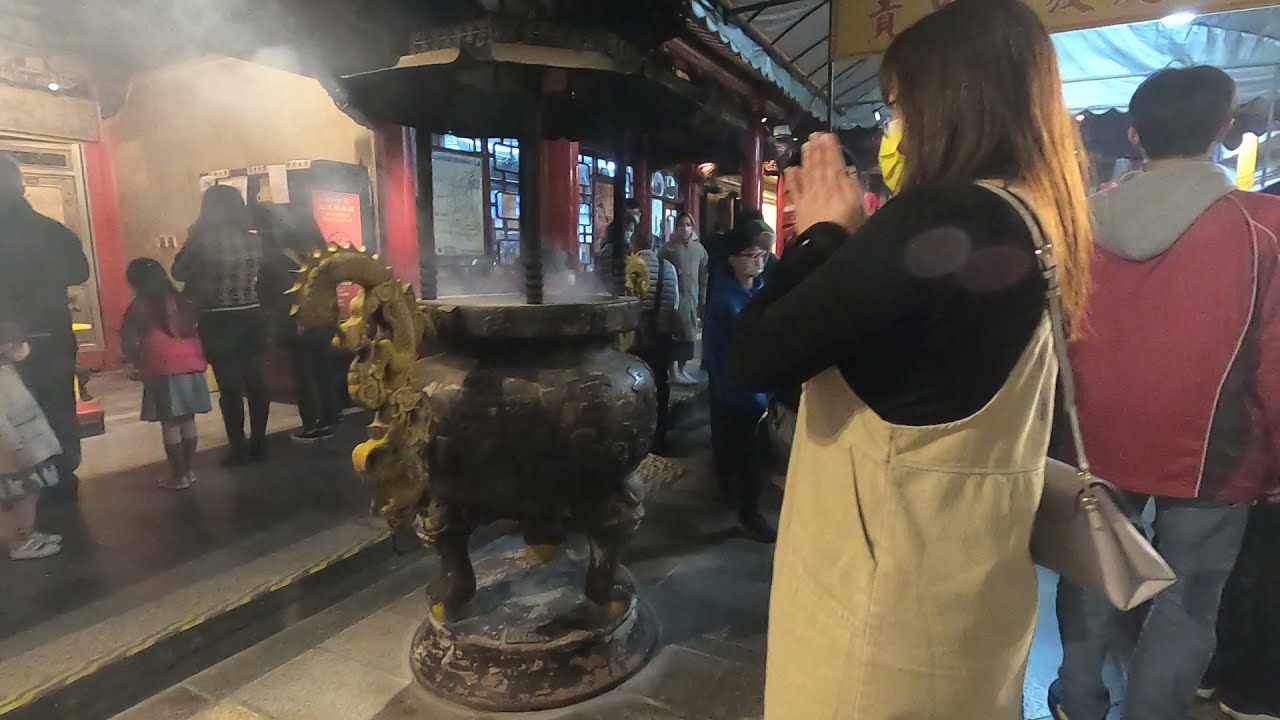In the image, an Asian woman is prominently situated on the right side, with her hands folded in a praying gesture. She is facing a central statue, which features distinctive Asian art, including a yellow dragon and a pot with four supports from which smoke or steam is rising. This statue is the focal point in the middle of the scene. Surrounding the central figure, several other people can be seen walking around, seemingly exploring the area and looking at various other statues, posters, and objects throughout what appears to be an indoor setting. The environment looks like an atrium, possibly part of a mall or in front of an Asian restaurant, judging by the decor and presence of multiple Asian individuals. The colors featured in the image include tan, black, yellow, brown, red, blue, and gray. Although there are banners in the background that appear to have Asian script, the text is not readable in the image.